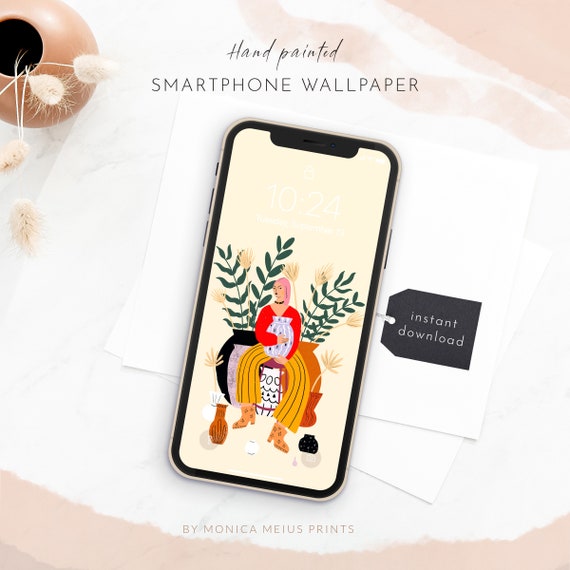The advertisement showcases a hand-painted smartphone wallpaper available for instant download, created by Monica Mia's Prints. The scene is a photograph of a desk-like surface with a few sheets of paper and a tan pot featuring dried flowers in the upper left corner. The main focus is a smartphone displaying the wallpaper, which depicts a woman sitting on a purple stool. She is hugging a vase and is surrounded by larger vases with lush plants. At her feet are two cats, one orange and one black. The woman is dressed in short boots and striped pants. The vibrant artwork, set against a yellowish-tan background, is complemented by a black tag with white writing indicating the instant download option. The text "hand-painted smartphone wallpaper" is prominently displayed, emphasizing the unique, artistic nature of the product.